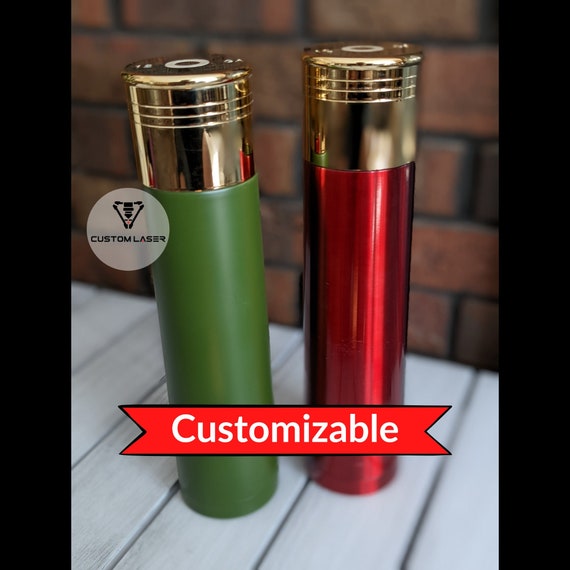The image captures a close-up view of two cylindrical objects that resemble vapes or bullet casings, each adorned with a gold cap. The cylinder on the left features an opaque green color, while the one on the right boasts a metallic reflective red surface. Both cylinders rest on a wooden table painted white, set against a background of orangey brick with black grout. Below the cylinders, a bright red ribbon prominently displays the word "Customizable" in white text. To the left of the cylinders, a small circle appears, containing the text "Custom Laser" in black, alongside an inverted triangular symbol. The intricate composition of the photograph highlights the contrasting colors and textures of the objects against the rich, textured background.